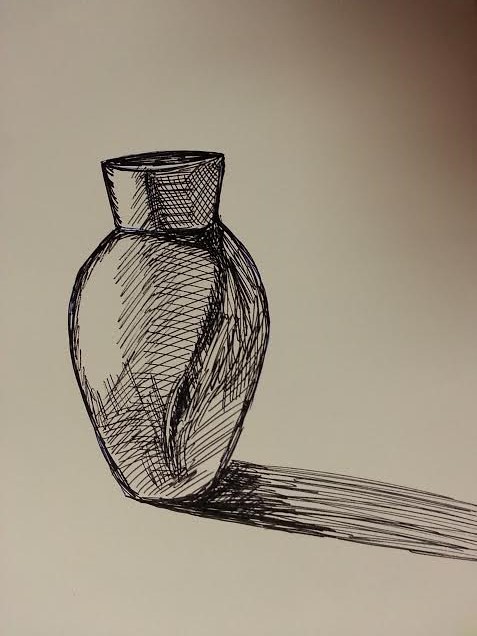A meticulously detailed pen and ink sketch graces a tan background, showcasing a traditionally shaped vase positioned on the left side of the image. The top left side of the vase reveals a clear tan coloring, untouched by pen highlights, suggesting a source of light from that direction. In contrast, the right side and bottom of the vase, along with the rim around the top, are adorned with numerous diagonal lines and areas of denser, darker scribbles. These intricate lines and textures masterfully depict the play of shadow and light enhancing the vase's form. On the bottom right of the vase, a subtle diagonal band of straight pen lines extends towards the edge of the image, representing the shadow cast by the vase due to the light source from the left.